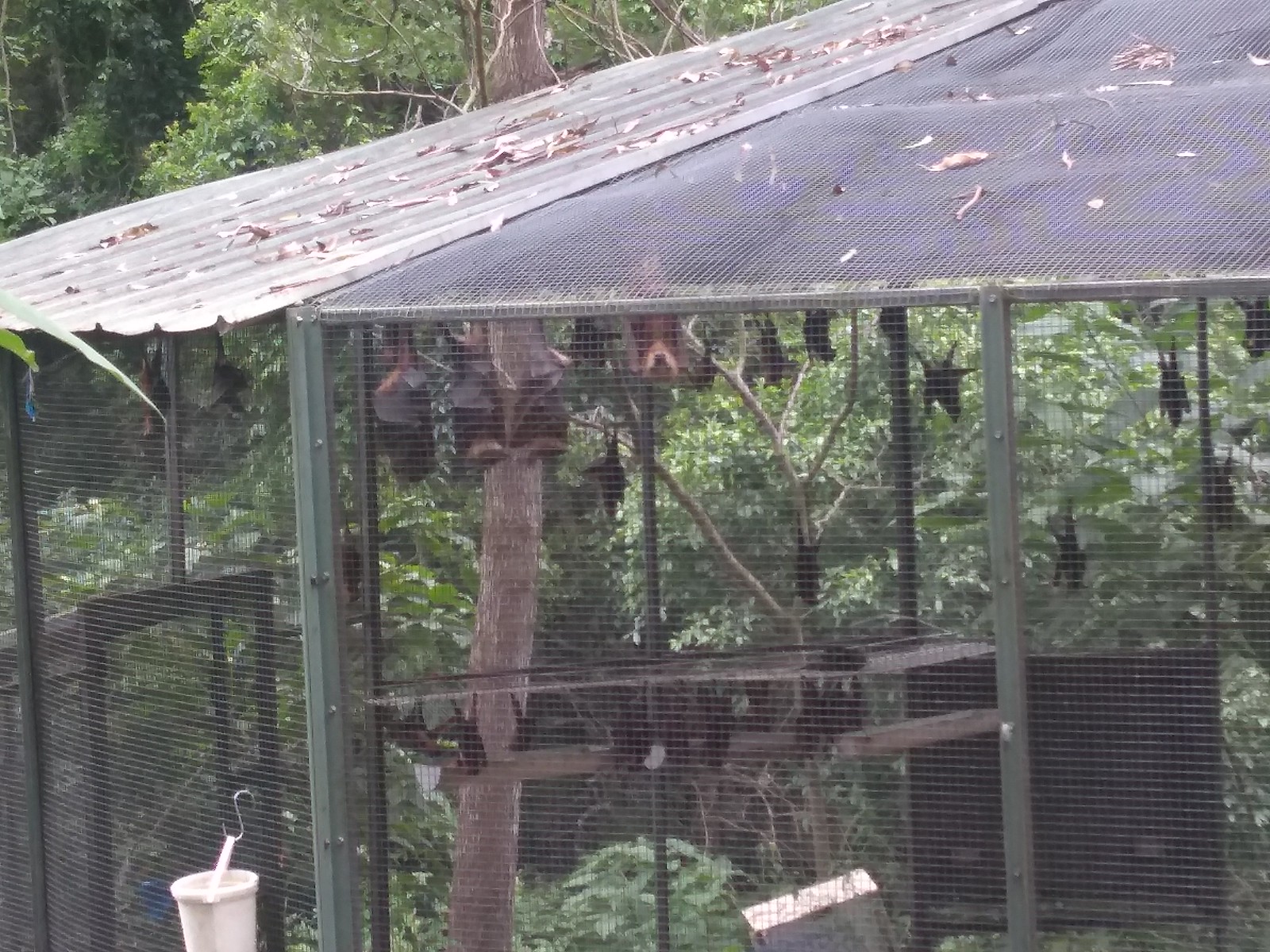This is a landscape-oriented, color photograph depicting an outdoor zoo enclosure designed as an aviary. The structure is predominantly covered in fine chicken wire mesh, including the front and a section of the roof, while another portion of the roof features corrugated sheet metal. The enclosure is supported by metal and wooden posts and contains multiple bats, which are either black or brown in color. These bats are seen hanging upside down from the wire mesh ceiling, from branches, and from various holders suspended within the enclosure. Within the left part of the image, a tree branch extends into the aviary, contributing to the naturalistic setting. Outside the enclosure, there are visible trees and greenery, adding depth to the background. In the bottom left corner of the image, a white disposable cup with a straw is situated, likely atop a table, near a bucket attached to the chicken wire with a silver s-shaped hook. Scattered dried brown leaves contribute to the scene atop the roof, emphasizing the outdoorsy environment. There are no people or motorized vehicles in the photograph.